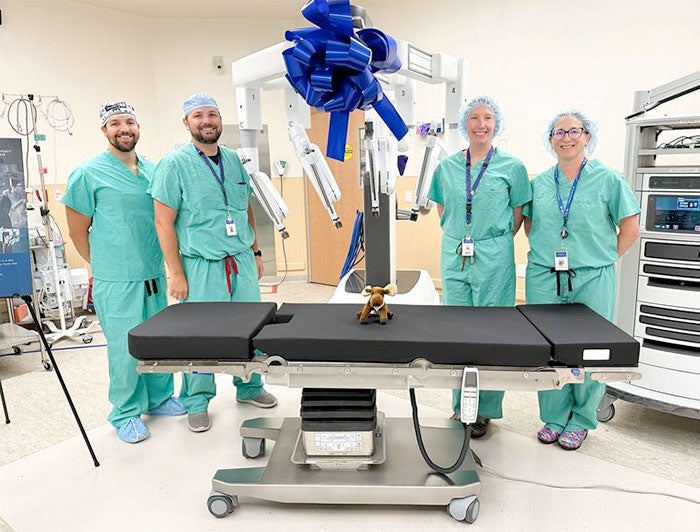The image captures an operating room inside a medical facility with an empty, adjustable operating table prominently in the foreground. This table features a black foam surface segmented into three parts—head, body, and feet—mounted on a stainless steel frame with black rungs for height adjustment, and resting on a wide footplate with dual-colored grey wheels. A silver remote control with a black cable is visible, attached to the table. Notably, a small brown stuffed moose lies atop the table. Towering behind the table is an elaborate grey and white robotic surgical apparatus, adorned with a large blue bow, indicating it might be a newly acquired piece of equipment.

In this celebratory scene, four medical staff members stand proudly on either side of the robotic machine—two men on the left and two women on the right—all dressed in green surgical scrubs and blue hairnets. Some wear blue shoe covers and ID lanyards, though these details are slightly blurry. The men, both bearded and appearing as twins, have differing postures; one stands with arms behind his back, the other with arms by his side. The women, standing side by side, also have their arms behind their backs. The backdrop reveals additional medical instruments, including drip stands and an equipment trolley with drawers and monitors, all on wheels. The room's beige and grey-speckled flooring contrasts with its off-white walls and ceiling, with a partially obscured, beach-colored door in the background. This image encapsulates the triumphant moment of unveiling a new piece of medical technology amidst an array of standard operating room equipment.